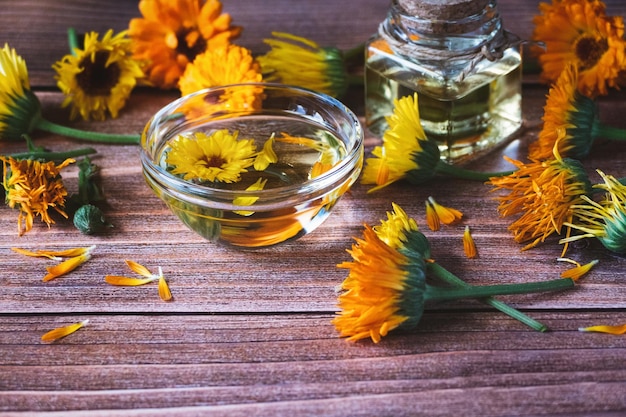The photograph captures a rustic, autumn-themed scene centered around nature's beauty. Atop a dark brown, unstained wooden table with visible horizontal wood grain, a clear glass bowl filled with water holds a small sunflower head accompanied by loose sunflower petals floating on the surface. Scattered across the table are numerous sunflower blossoms, varying in shades of yellow and orange, with some appearing freshly picked while others seem dried. These sunflowers include different varieties, distinguished by varying petal widths and seed head sizes. Adjacent to the bowl is a square glass jar with a cork top containing a yellow liquid, potentially related to the sunflowers. The overall image evokes a serene, fall atmosphere, with the sunflowers' vivid colors contrasting beautifully against the natural, rustic wooden background.